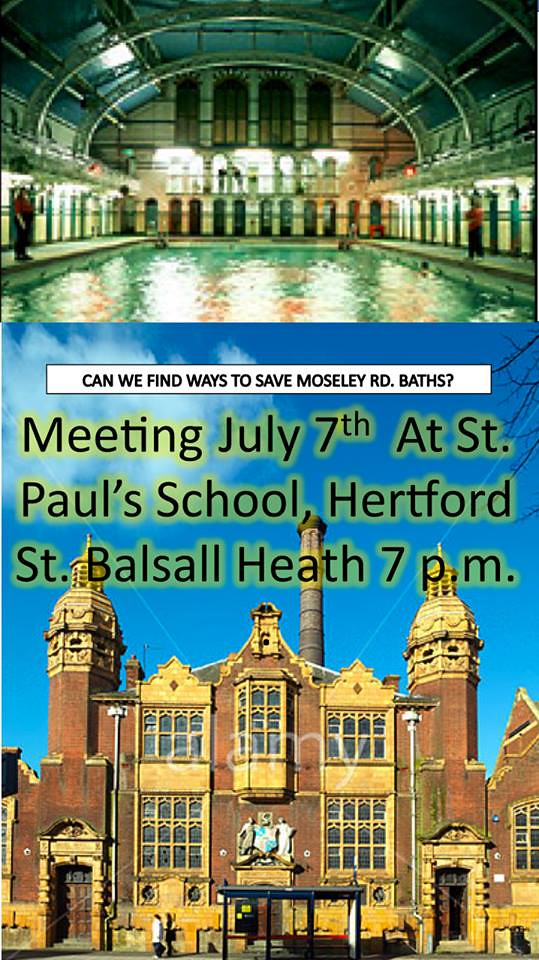The image comprises two color photographs in a portrait orientation. The top photograph features the interior of an indoor swimming pool facility with a large arched glass roof. This portion is slightly blurry and appears to show two coaches, one on the left and one on the right, possibly overseeing swim practice. Superimposed on this image is a prominent sign with black text on a white background that reads, "Can we find ways to save Moseley Road baths?"

Beneath this is a clearer, more detailed photograph of the exterior of an ornate, old-fashioned building made of terracotta and gold-colored materials, with life-size statues on the wall. The building has two towers on either side and elaborate gables over windows. Additional text overlaid on this photograph, in larger black letters with a yellow drop shadow, announces an event: "Meeting July 7th at St. Paul's School, Hertford St. Balsall Heath, 7 p.m." The sky in the background is a vivid blue, indicating a bright, sunny day.